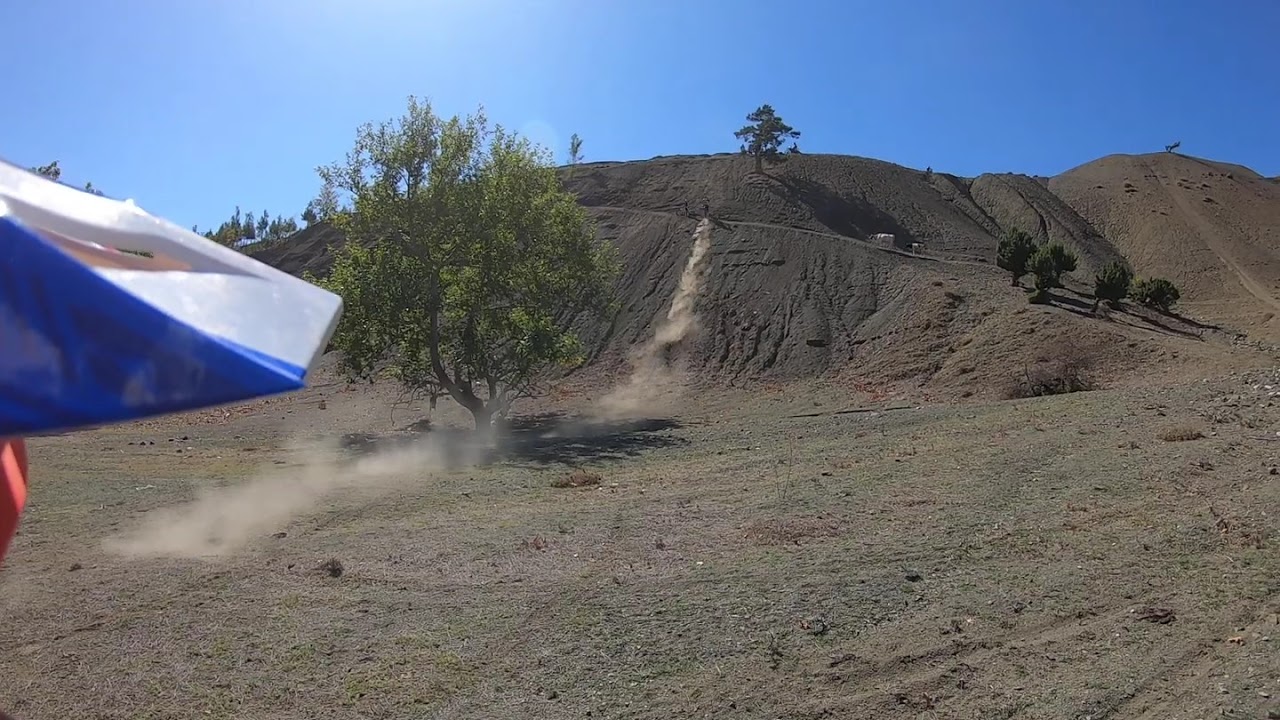The image showcases a vast, mostly barren landscape under a clear, light blue sky, possibly taken in the middle of the day. The terrain is hilly and desert-like, featuring a large, open grass and dirt field spanning the foreground. A roadway cuts through the landscape, with visible tracks suggesting recent activity, likely from an ATV or motorcycle. An individual on a vehicle is climbing a hill, leaving a trail of dust clouds. Scattered across the property are sparse shrubs and evergreen trees. On the ridgeline, several trees can be seen, with one larger tree standing prominently atop a hill. In the left part of the picture, a partially visible triangular structure, possibly an umbrella with red, blue, and white sections, provides a splash of color and shade. A puff of dust near this structure hints at recent movement. Some hills and distant mountains accentuate the background, bathed in a beautiful, clear blue sky. The scene epitomizes a rugged, outdoor setting, highlighting nature's raw and expansive beauty.